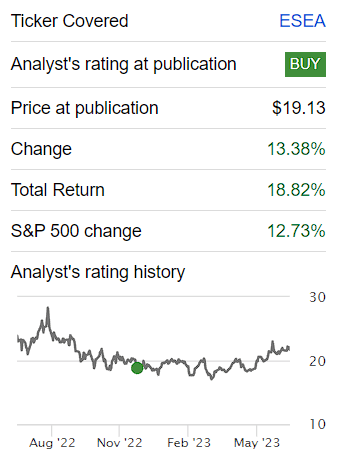The image appears to be a structured screenshot with a white background, divided into seven rows separated by thin, light gray lines. Each row contains black text on the left and various elements on the right. Here's a detailed breakdown:

1. The first row has the label "Ticker Covered" on the left and, on the far right, the ticker symbol "ESEA" displayed in bold blue capital letters.
2. The second row is labeled "Analysts Rating at Publication" and features a green rectangular box with the word "Buy" in white letters to its right.
3. The third row, labeled "Price at Publication," shows the figure "$19.13" to its right.
4. The fourth row is titled "Change" and displays "13.38%" in green.
5. The next row is labeled "Total Returns," with "18.82%" in green to its right.
6. The sixth row reads "S&P 500 Change" and lists "12.73%" on the right.
7. The final row, "Analysts Rating History," features a gray graph ranging from August 2022 to May 2023. The x-axis marks August 2022, November 2022, February 2023, and May 2023, while the y-axis ranges from 10 to 30. A green dot is visible on the graph, indicating a specific data point.

This detailed description captures the structure and content of the screenshot accurately, including the text, numerical data, graphical elements, and color scheme.